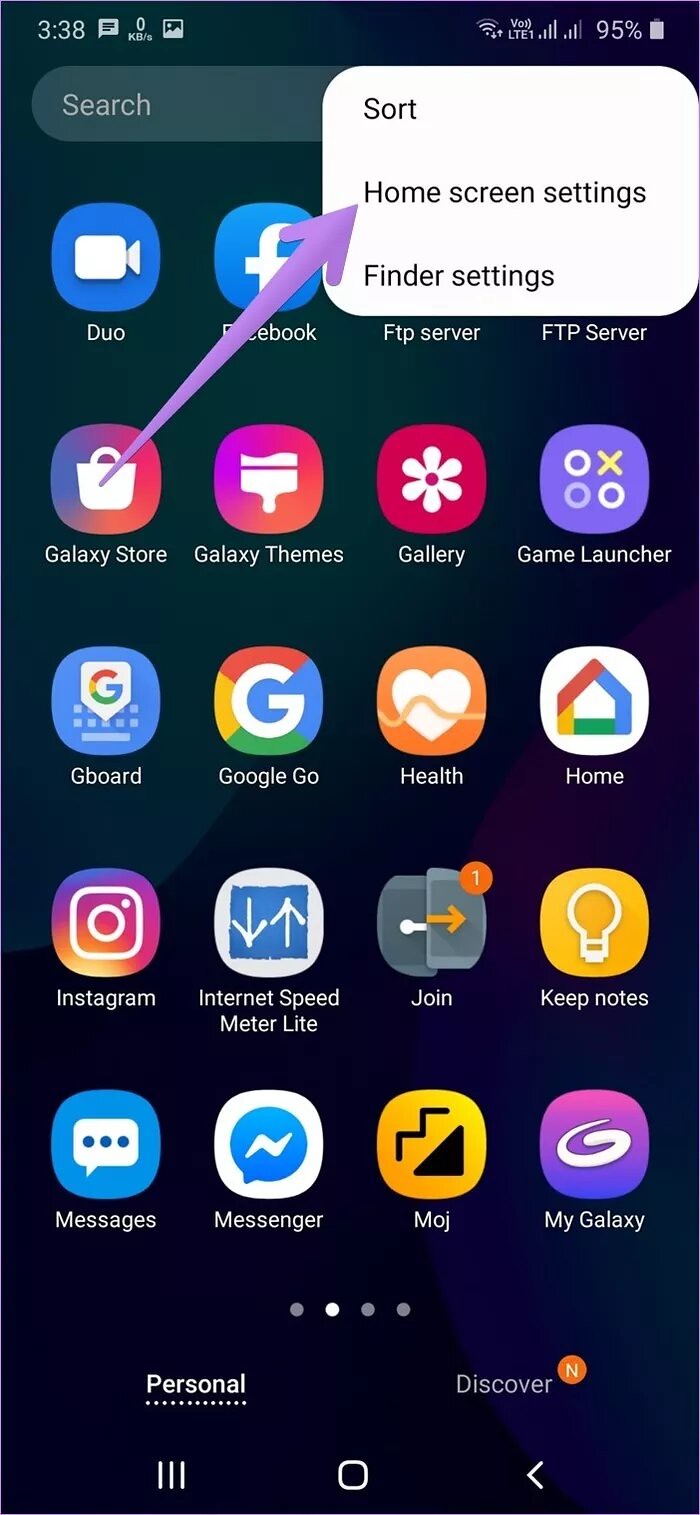This screenshot captures the second page of a smartphone's dashboard with a minimalist black background. At the top, there's a search bar and the battery icon indicates a 95% charge level. The middle section features an active Galaxy Store update highlighted by a purple arrow at a 45-degree angle pointing to a white pop-up menu with options labeled “Sort,” “Home Screen Settings,” and “Finder Settings.” The apps arranged in a grid format include Google Go, Home, Gallery, Galaxy Themes, Gboard, Instagram, Keep Notes, My Galaxy, Messenger, and Messages. Additionally, there are apps named Modge, John, Internet Speed Meter Lite, and another instance of Keep Notes displayed. The current time shown on the screenshot is 3:38 PM.